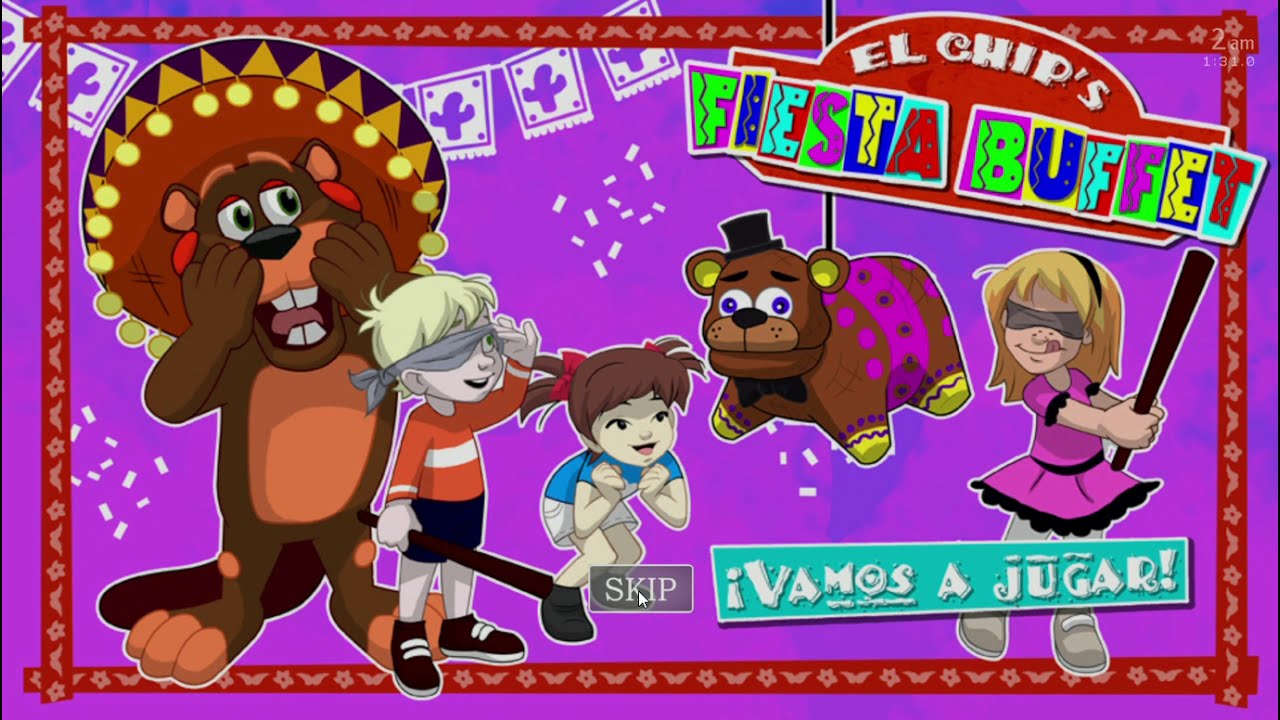The image is a vibrant and densely detailed illustrated banner with a bright purple background and bordered with a red trim. At the center, three children—two girls and one boy—are gathered around a piñata resembling a teddy bear with a top hat, which strongly hints at a connection to the game "Five Nights at Freddy's." The boy, who is peeking out from under his blindfold, grips a stick in his hand, while one girl crouches excitedly with pigtails sticking out, and the other girl positions herself to hit the piñata with her own stick, blindfolded. To the left of the children stands a cartoonish beaver character wearing a sombrero, his hands to his cheeks and mouth open as if in shock. At the top right of the image, bold text reads "L Chips Fiesta Buffet" in colorful, playful letters, and at the bottom right, a banner with the Spanish phrase "¡Vamos a jugar!" emphasizes the festive, animated theme. The image is filled with an array of colors including pinks, blues, reds, greens, peaches, browns, and light blues, contributing to the lively, celebratory atmosphere. A "skip" button at the bottom center indicates that this might be a menu screen for a game.